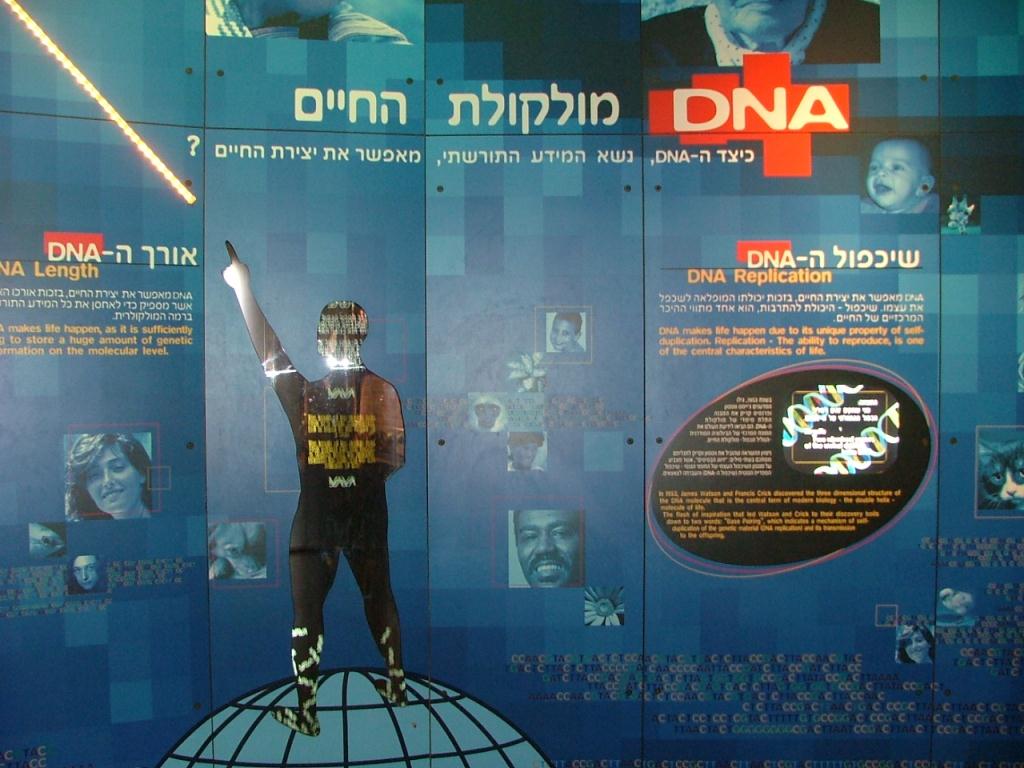The image appears to be a science exhibit focused on DNA, prominently featuring blue as the background color, composed of smaller squares in varying shades of blue that create a manifold effect. The predominant text is mostly in Hebrew, with some in English, and includes orange and white lettering that reads "DNA replication" and "DNA" respectively. Towards the top right, DNA appears again in white letters against a red geometric background. On the left side, though not the extreme left, stands a silhouette of a person dressed in black, pointing upwards, atop a light blue, artistically rendered globe. Surrounding this are numerous monochromatic images, primarily in blue hues, of different people's faces. The exhibit includes additional written information, though some details are small and difficult to read, including mentions of key concepts like DNA replication and DNA length.